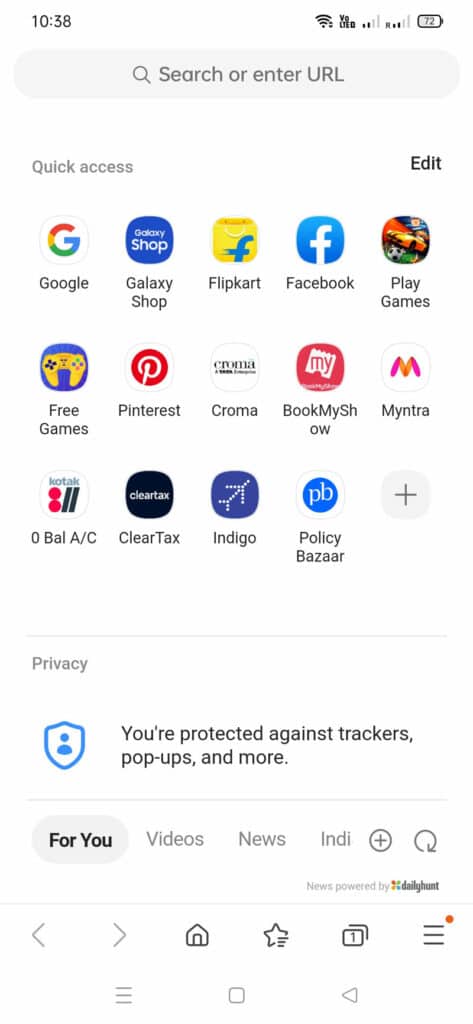Screenshot of an Android device showcasing the settings tab. At the top of the screen, the status bar shows the time as 10:38, with no indication of AM or PM. The status bar also displays the Wi-Fi signal strength, cell reception bars, and a battery life at 72%. 

Below the status bar, there's a prominent gray search bar with the text "Search or enter URL," designed for easy navigation within the device. The main section of the screen features three rows of five application icons each, totaling 15 app icons. Prominent apps include Google, Galaxy Shop, Flipkart, Facebook, and Play Games among others.

Near the bottom of the screen, there is a single icon, a plus symbol, likely for adding more applications. Beneath this grid of icons, a segment of the privacy settings is partially visible, displaying a message about protection against trackers and pop-ups. 

Additionally, at the very bottom of the screen, there is a navigation menu with tabs labeled "For You," "Videos," "News," and "Indy," alongside another plus icon for presumably adding or customizing content.

The layout and app selection strongly suggest this is an Android device, further reinforced by the presence of numerous Google-related apps and services.